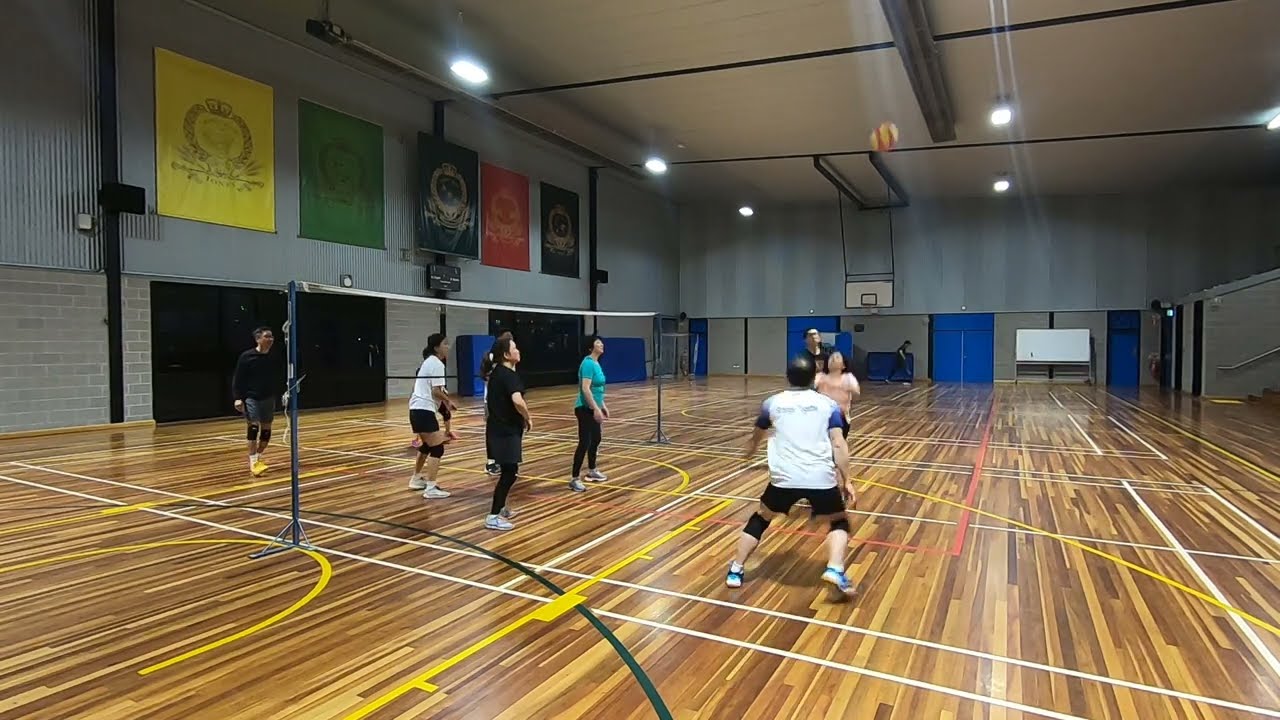The photograph captures a lively moment inside a gymnasium, where a spirited volleyball game is underway on a hardwood basketball court. The court is marked with various colored stripes and tapes for different sports. Prominently featured in the center of the action, a man wearing knee pads, a white and blue shirt, and black shorts, and a girl in a pink shirt are both leaping towards a red and yellow volleyball, which is caught mid-air in motion blur. The volleyball net, supported by two blue poles, clearly segments the court. High on the far wall, five large banners in yellow, green, blue, red, and black display distinctive crests. Overhead, bright ceiling lights illuminate the entire scene, and there's visible padding around certain areas of the gym. Toward one side, a set of steps leads down to the main court area, and several doors are also noticeable along the walls. The photograph beautifully captures the vibrant atmosphere and intensity of the game.